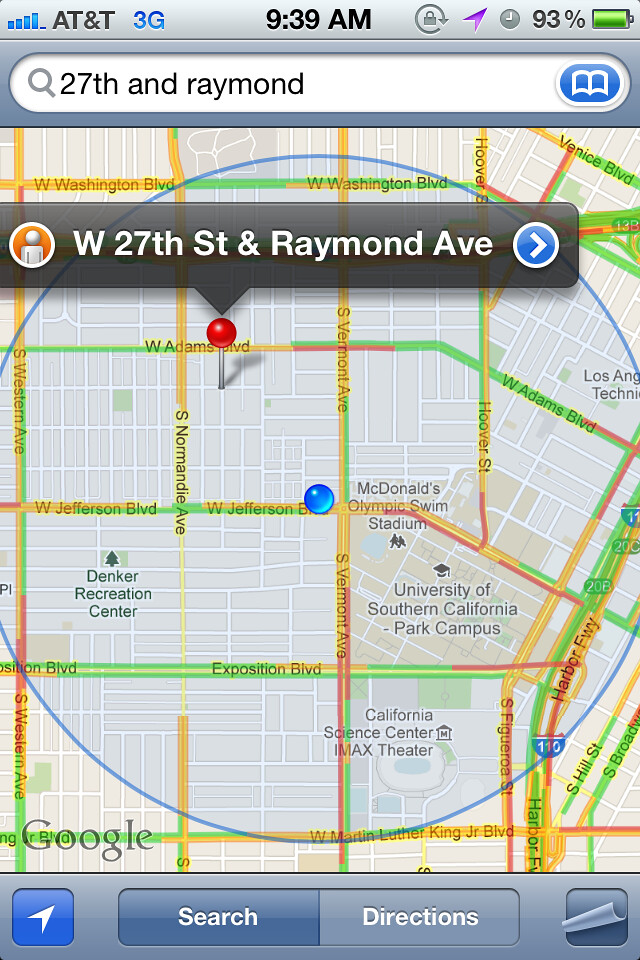This image is a detailed screenshot of a Google Maps display on a cell phone screen, showcasing the map around the intersection of 27th Street and Raymond Avenue. The phone, subscribed to AT&T, displays a variety of status icons at the top: AT&T service in black text, a blue "3G" indicator, the current time "9:39 AM" in black, a gray circular arrow with a lock, a purple navigation pointer, a white clock icon, "93%" battery life in black text, and a green battery icon.

Below these status icons is a search bar displaying the query "27th and Raymond," featuring a blue oval icon with a white open book symbol. 

The map itself presents a dark gray translucent rectangle overlay with white text indicating "W 27th Street and Raymond Avenue." On the left of these words is an orange circle framed in white with a white person icon, and on the right is a blue circle framed in white with a right-pointing white arrow icon.

A push pin marks the searched location on the map, which shows surrounding city streets with traffic conditions highlighted in green, yellow, and red, indicating varying levels of traffic congestion. Points of interest on the map include the University of Southern California Park Campus and nearby McDonald's Olympic Swim Stadium. Further south on West Martin Luther King Jr. Boulevard are additional landmarks such as the California Science Center and the IMAX Theater.